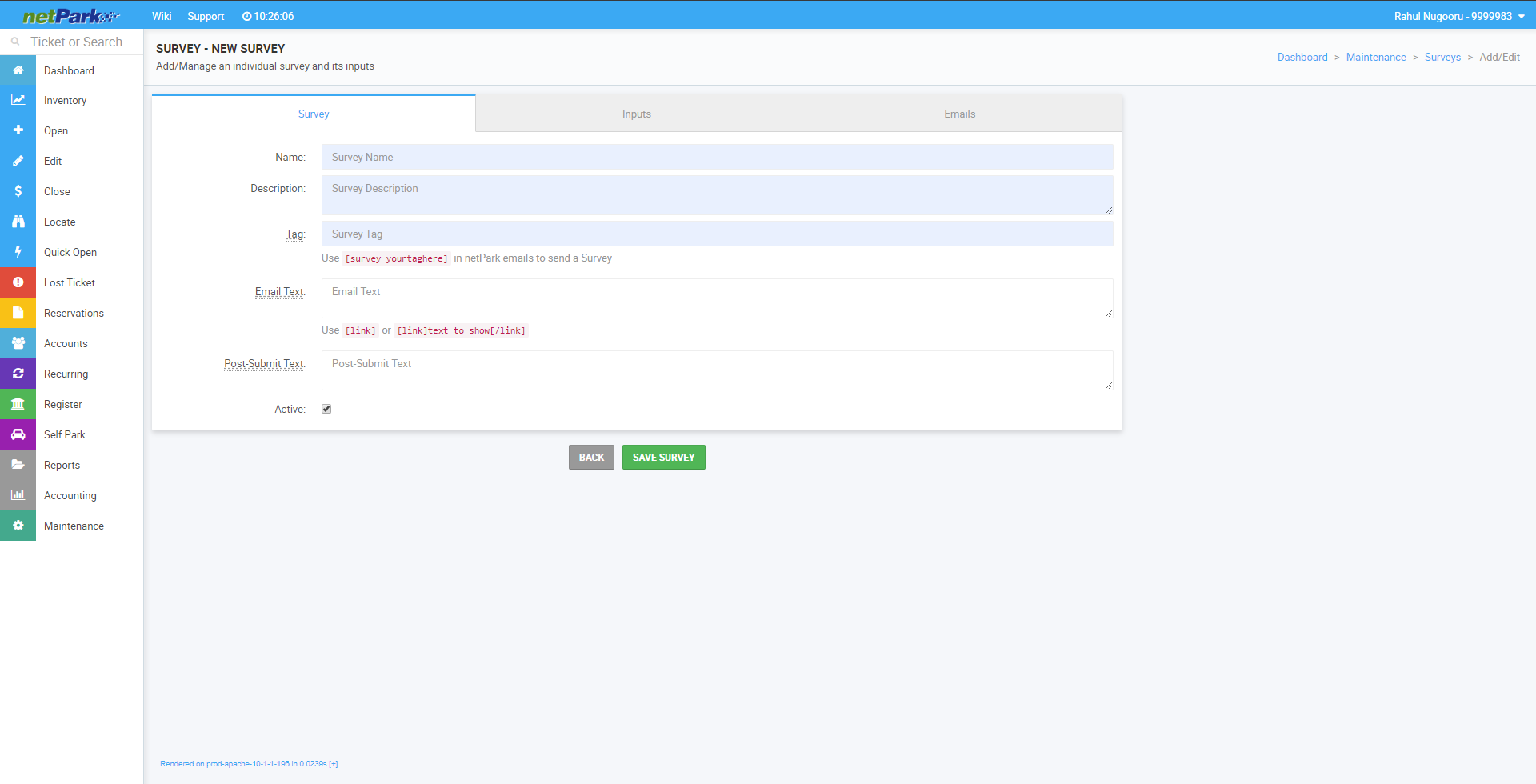This screen capture displays a computer monitor featuring a layout for a Wiki Support ticket management system. A top banner in cornflower blue spans the width of the screen, with the left side displaying the label “NET” in a grey-green lowercase font and “PARC” in dark blue letters with a capital 'P'. On the right side of the banner, the white text reads “Wiki Support” and “1026.06”.

Running vertically along the left side of the screen is a long rectangular window with a search bar at the top saying "Ticket or Search". This section also contains a partial upper left blue banner accompanied by a set of menu options with icons in white to the left of each label. The menu items include:

- Dashboard
- Inventory
- Open
- Edit
- Close
- Locate
- Quick Open

Below these items, there are additional coloured squares with further options, each with corresponding icons:
- Orange: Lost Ticket
- Yellow: Reservations
- Blue: Accounts
- Purple: Recurring 
- Green: Register
- Purple: Self-PARC
- Grey: Reports
- Grey: Accounting
- Green: Maintenance (the last menu item)

In the central section on the right, the top-left corner of the window has text in black reading "Survey, new Survey." Below this, in black lettering, it says "Add Manage an Individual Survey and its Inputs." The main tab displayed is "Survey" in blue on a white background. Beneath this header are three lines labeled "Name", "Description", and "Tag", each with an adjacent text box for input. Further down, there are another two text boxes labeled "Email Text" and "Post Submit Text". Adjacent to "Active" is a checked checkbox. Up top, there are two additional background tabs labeled "Inputs" and "Emails".

At the bottom of the form, there are two buttons: a grey button on the left labeled "Back" in white lettering, and a green button on the right labeled "Save Survey" in white lettering.